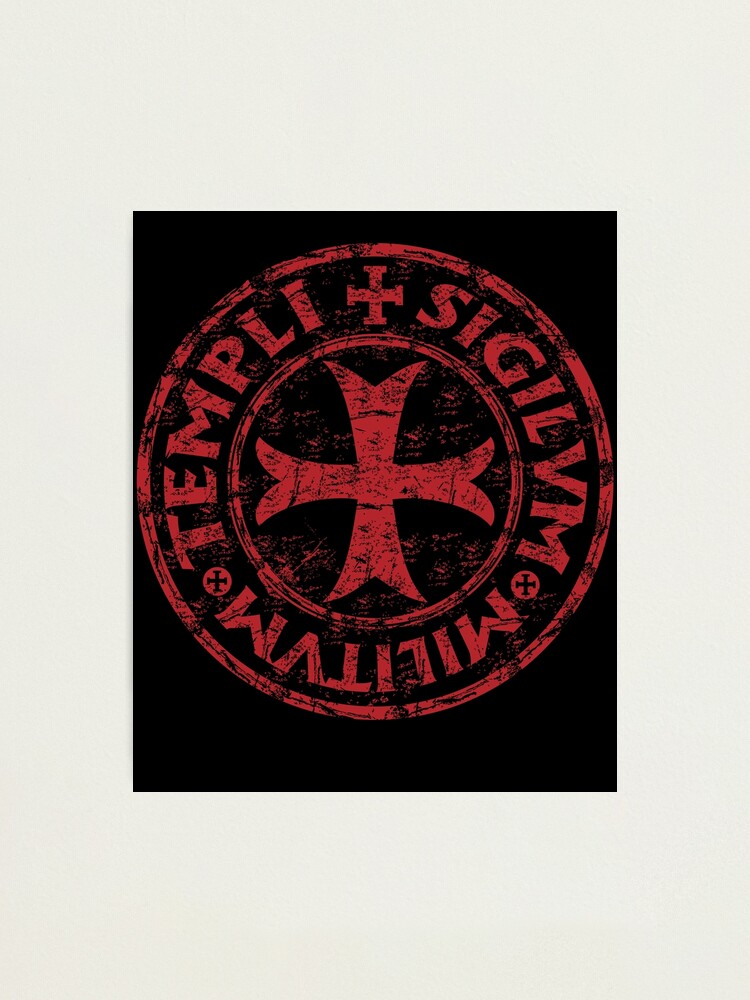The image depicts a striking black graphic heavily bordered by off-white, extending to the edges of the image. Central to the graphic is a weathered and grungy red circle, which features both an outer and inner ring with text around the circumference. The text, appearing to be in Latin, reads "TEMPLI SIGILVM MILITVM," surrounding a large red cross centrally positioned in the inner circle against a black background. This cross has a slightly angled and rounded design at the top and bottom edges, with the entire circular motif resembling an old sign or seal. The outer red ring of the circle, embellished with cuts, scratches, and faded textures, adds an antiquated and militant appearance possibly reminiscent of medieval or biker iconography, such as a Knight Templar seal. The overall aesthetic is gritty, combining stark red and black on a predominantly white border, making it a compelling and enigmatic visual that invites further interpretation.